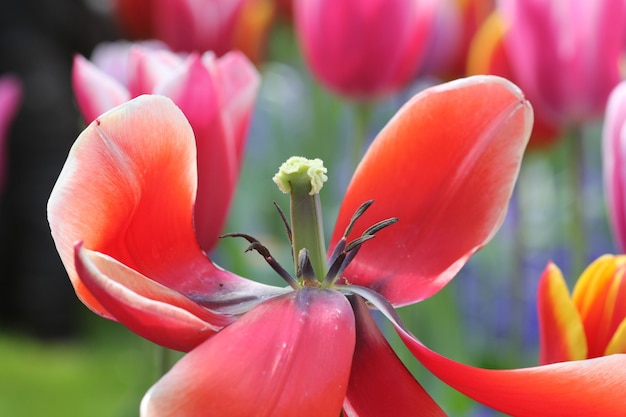This photograph features an up-close, horizontally oriented view of a tulip that's beginning to fall apart. The flower’s petals transition from a deep red or dark orange at their bases to a lighter, almost white, hue at the edges. The center of the tulip showcases a prominent green pistil, topped with a nearly white, fluffy substance where the pollen is held. Surrounding the pistil are dark brown, almost black, spiky anthers radiating outward. In the blurred background, several other tulips can be observed, primarily pink with white tips and a few showcasing orange and yellow tones. To the lower right, there is a distinctly visible orange-and-yellow tulip bud. The backdrop of the image transitions from black at the upper left to green at the lower left, possibly indicating grass or foliage.